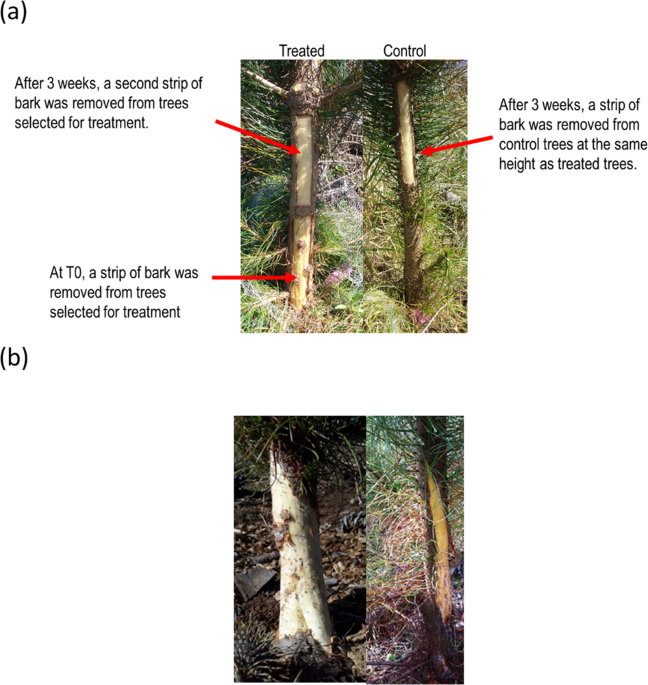The image consists of two sets of side-by-side photographs labeled A and B, each comparing tree trunks under different conditions. 

In section A, the photographs highlight the effects of bark removal on tree trunks over a three-week period. The left image is labeled "treated" and depicts the treated tree trunk with annotations: a red arrow at the lower part indicating where a strip of bark was removed initially (T0) and another red arrow at a higher point marking the second strip removed after three weeks. The right image, labeled "control," shows the control tree trunk with a red arrow pointing to the area where a strip of bark was similarly removed after three weeks, at the same height as the treated tree. Text details emphasize the timing and procedure of bark removal for both treated and control trees.

In section B, the comparison shifts to the visual differences in tree trunks' appearances. The left trunk exhibits a stark white color, while the right trunk is characterized by a yellowish hue. This section further illustrates the physical impacts of the treatments over time.

Overall, the image serves as a detailed comparison between treated and control trees, demonstrating both the procedural aspects and the resulting changes in trunk appearance.